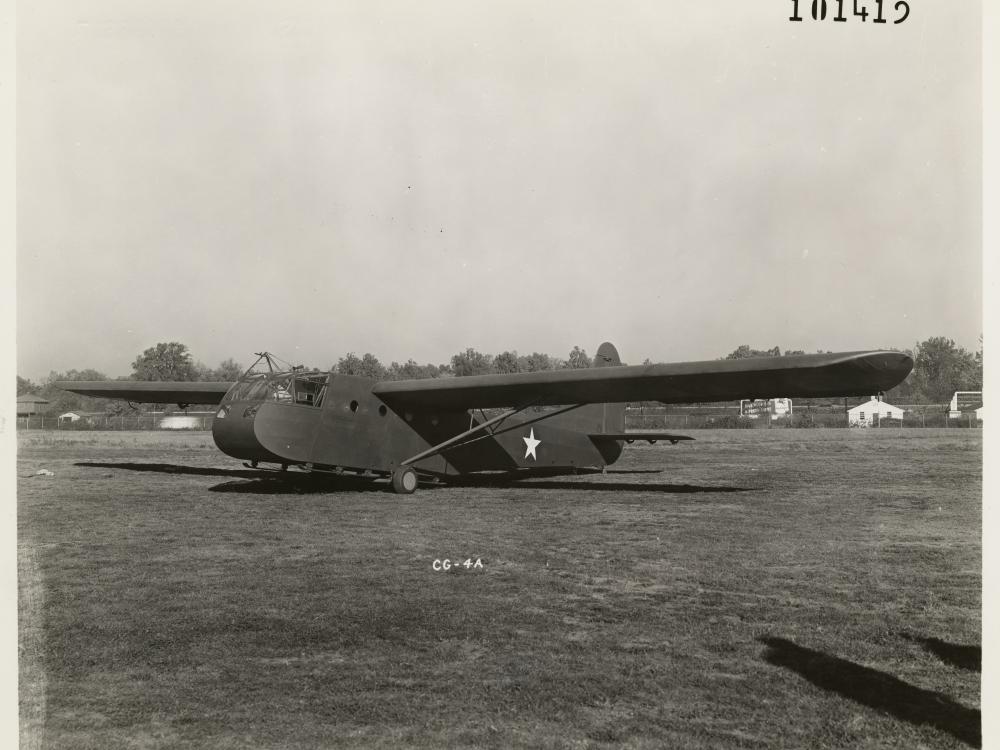In the black and white photograph before me, the focal point is a vintage airplane, seemingly a relic from an era just post-World War I. The aircraft's design is markedly simplistic and bare, composed primarily of sheet metal and exhibiting minimal cover or additional attachments. It does not boast any advanced or elaborate features, with no visible gunner seat or armament, suggesting it might have been an early prototype or a less developed model. This minimalistic design gives an impression of cost-effective and rapid production, possibly indicating it was an experimental or transitional model in aviation history.

A notable detail supporting its military origins is a faint, white star visible on the left-hand side of the aircraft's fuselage, a classic emblem of the U.S. military. The plane's overall structure is utilitarian, with its boxy shape emphasizing function over form. This photograph offers a fascinating glimpse into early military aviation and the evolutionary steps leading up to more sophisticated designs.